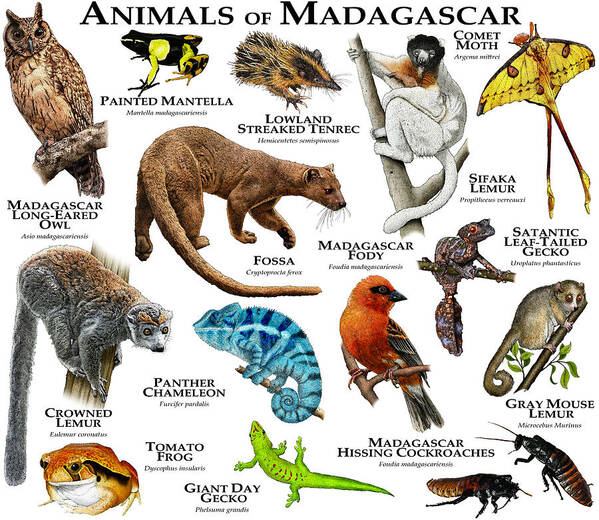This detailed poster showcases the fascinating diversity of Madagascar's wildlife against a clean white background with striking black capital letters spelling out "Animals of Madagascar." The meticulously illustrated collection features 15 distinct species, each with a descriptive title. Notable animals include the Madagascar Long-eared Owl, the vibrantly patterned Painted Mantella frog, and the lowland streak tenrec, which resembles a small rodent. The Comet Moth is depicted with its characteristic long tails, while the fossa, an elusive carnivore with cat-like and cougar-like features, adds an element of intrigue. The poster also highlights various lemurs, including the gray mouse lemur with its long, coiled tail and a typical lemur representative. Other remarkable creatures include a strikingly blue chameleon, the uniquely creepy Madagascar hissing cockroach, and the colorful Madagascar fatty, a bird that boasts orange and gray plumage reminiscent of an Oreo. Completing the array is the bizarre satanic leaf-tailed gecko. This visually rich guide serves as an educational overview of Madagascar's native fauna, offering a vivid snapshot of this island's unique ecosystem.